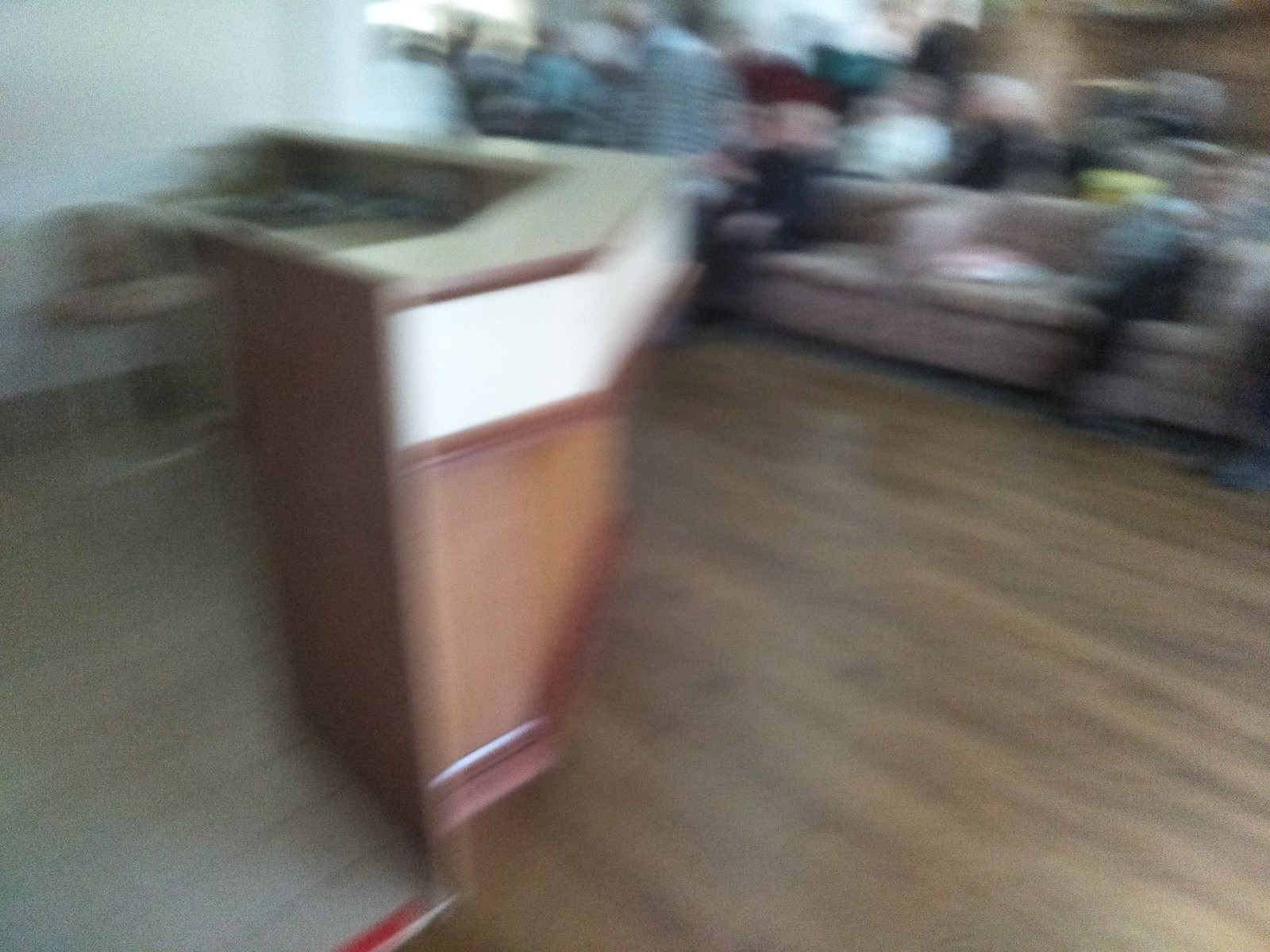In this highly blurred color photo of a public space, a large white and wood-colored podium with a red outline occupies the left half of the image. Behind the podium, a chair and a small shelf are visible, suggesting a reception desk, possibly in a small hotel or office. The floor near the podium is hardwood or vinyl, transitioning to white tiles on the left and a different, less discernible flooring. The right side of the photo features multiple couches or upholstered furniture in a beige fabric positioned along the top right corner. Numerous people, though very blurry, are crowded towards the back, some standing near windows, wearing varying colors—blue, red, green, and navy shirts. The room is brightly lit, but details are obscured due to the blurriness, making it challenging to determine specific activities or actions taking place.